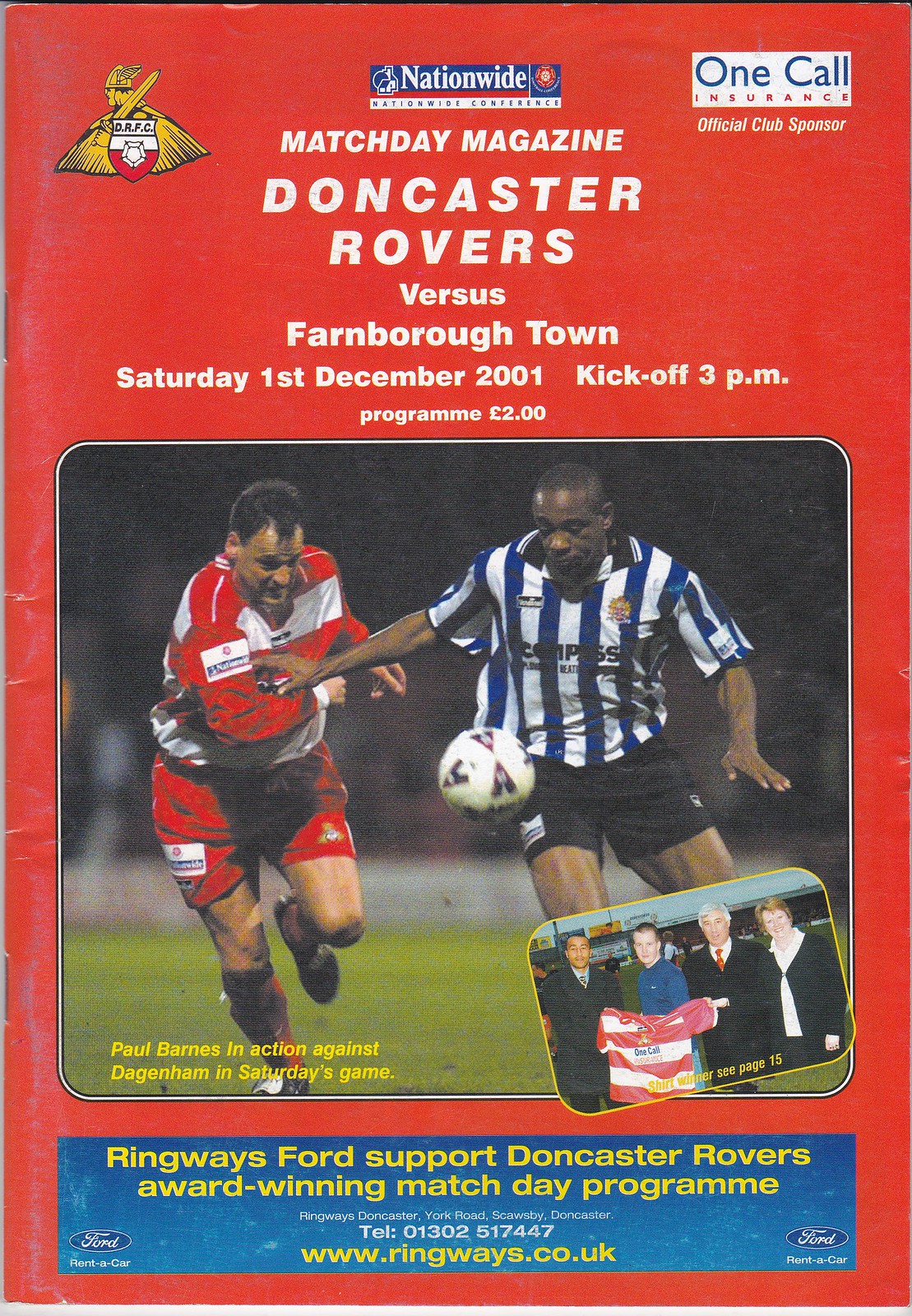The front cover of the Matchday Magazine for the Doncaster Rovers versus Farnborough Town, dated Saturday, 1st December 2001 with a 3 PM kickoff, prominently features striking visuals and comprehensive details. Dominated by a vivid red background, the upper section displays the Doncaster Rovers Football Club (DRFC) logo to the left, followed by logos for Nationwide and One Call Insurance, the official club sponsor. Below these logos, the title "Matchday Magazine" boldly announces the teams: Doncaster Rovers vs. Farnborough Town, emphasizing Doncaster Rovers' name in a larger font. Centrally, an action shot captures two players contesting the soccer ball, one in horizontal red and white stripes and the other in vertical white and blue stripes, with the ball levitating waist-high between them. One player is noticeably black, enhancing the dynamic scene. Superimposed below this is an image of four formally dressed individuals presenting a red jersey. Along the bottom, a blue banner, adorned with gold text, advertises, "Ringways Ford support Doncaster Rovers' award-winning match day program," along with the website, www.ringways.co.uk. The magazine is priced at £2.